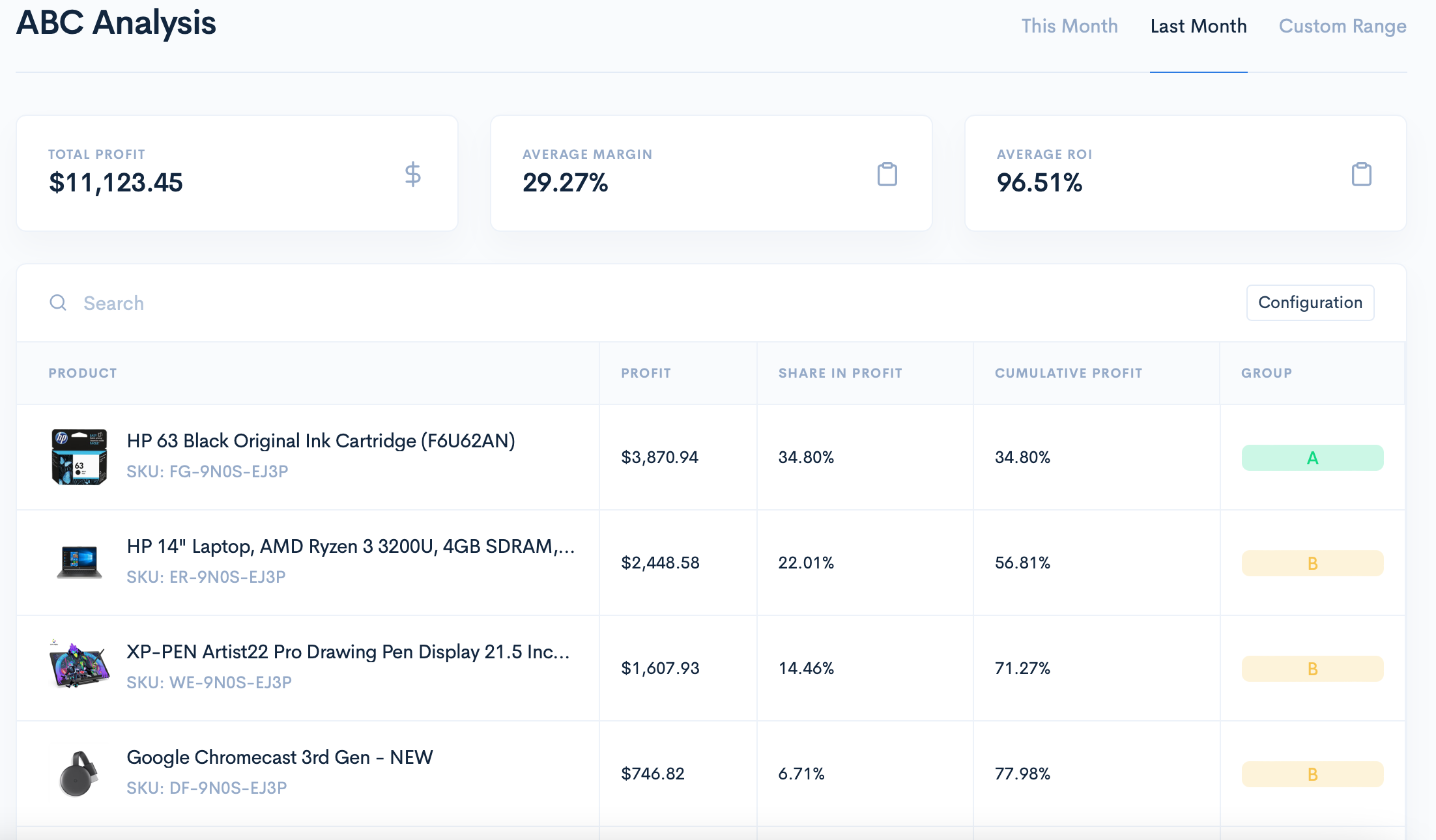This screenshot captures an ABC analysis tab displaying detailed metrics on product performance, specifically focusing on total profit, average margin, and average ROI. In the top right corner, there are options for selecting data ranges: "This Month," "Last Month," and "Custom Range," with "Last Month" currently selected. This selection is indicated by black text and a blue underline, while the other options appear in blue text.

At the top of the screen, three large white boxes present key financial metrics from last month:
1. **Total Profit:** $11,123.45
2. **Average Margin:** 29.27%
3. **Average ROI:** 96.51%

Beneath these metrics is a search bar that stretches across the full width of the screen. Below the search bar, the table headers list the following categories: Product, Profit, Share in Profit, Cumulative Profit, and Group. 

The first product listed is an HP ink cartridge, accompanied by a small thumbnail image. The associated financial data for this item is:
- **Profit:** $3,870.94
- **Share in Profit:** 34%
- **Cumulative Profit:** 34%
- **Group:** A

Three additional products are listed below the HP ink cartridge, following the same format of detailed financial metrics.